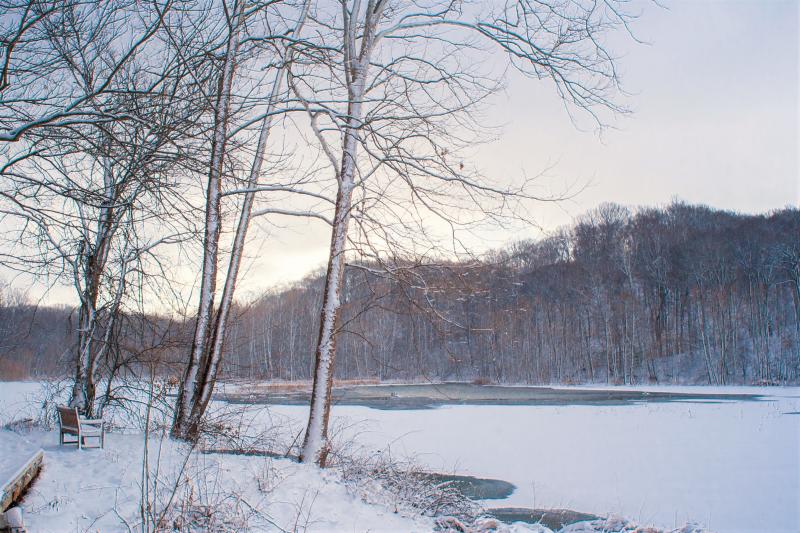The image captures a serene winter scene of a partially frozen lake, with snow and ice dominating the foreground. The lake features patches of open water where the ice has thawed, blending with the surrounding snow. On the lake's bank, a snow-covered wooden bench with backrest and armrests offers a tranquil viewing spot amidst the cold. Leaning, leafless trees with snow sticking to their trunks stand nearby on the left side, framing the bench. Dry grass pokes through the snow, adding texture to the wintry landscape. Across the lake, a tall tree line stretches from left to right, bearing the same barren and snow-dusted appearance. The distant hillside echoes this wintery feel, devoid of leaves but rich in seasonal details. The sky above is subtle, with the early morning light casting a very light orange hue, enhancing the peaceful ambiance of the winter wonderland.